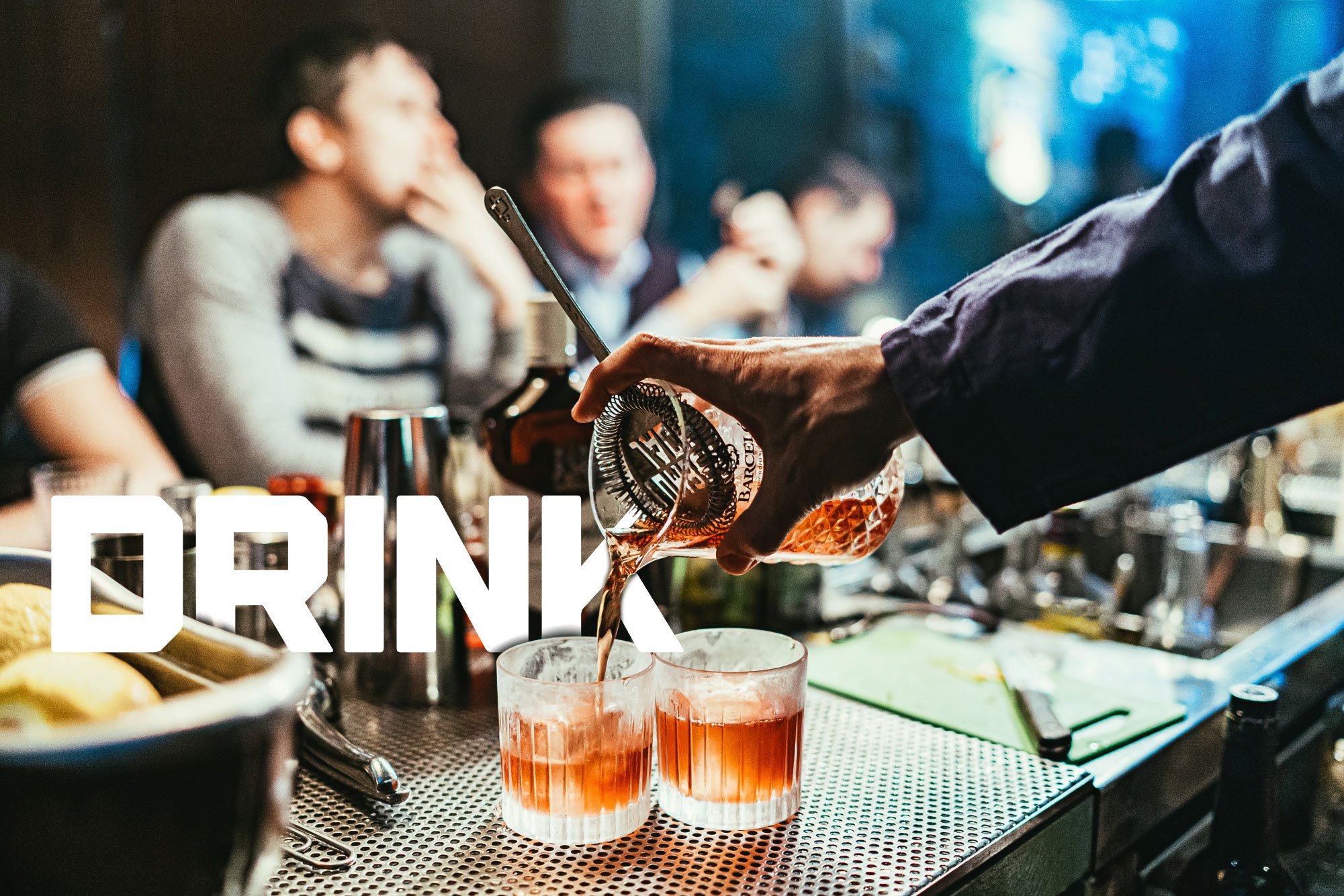The image depicts a lively bar scene with a male bartender dressed in a long-sleeve shirt meticulously preparing drinks. He is shown straining a reddish-brown cocktail into two frosted shot glasses, making sure to keep seeds or fruit bits out. The strainer has the word "DRINK" prominently displayed in large white letters. On the left side of the bar, there's a bowl of bread, a cutting board with a knife, and fresh lemons — suggesting preparations for additional garnishing. In the background, three or four indistinct figures can be seen, their slightly blurred forms indicating they are engrossed in conversation or other activities, adding to the bustling atmosphere of the bar.